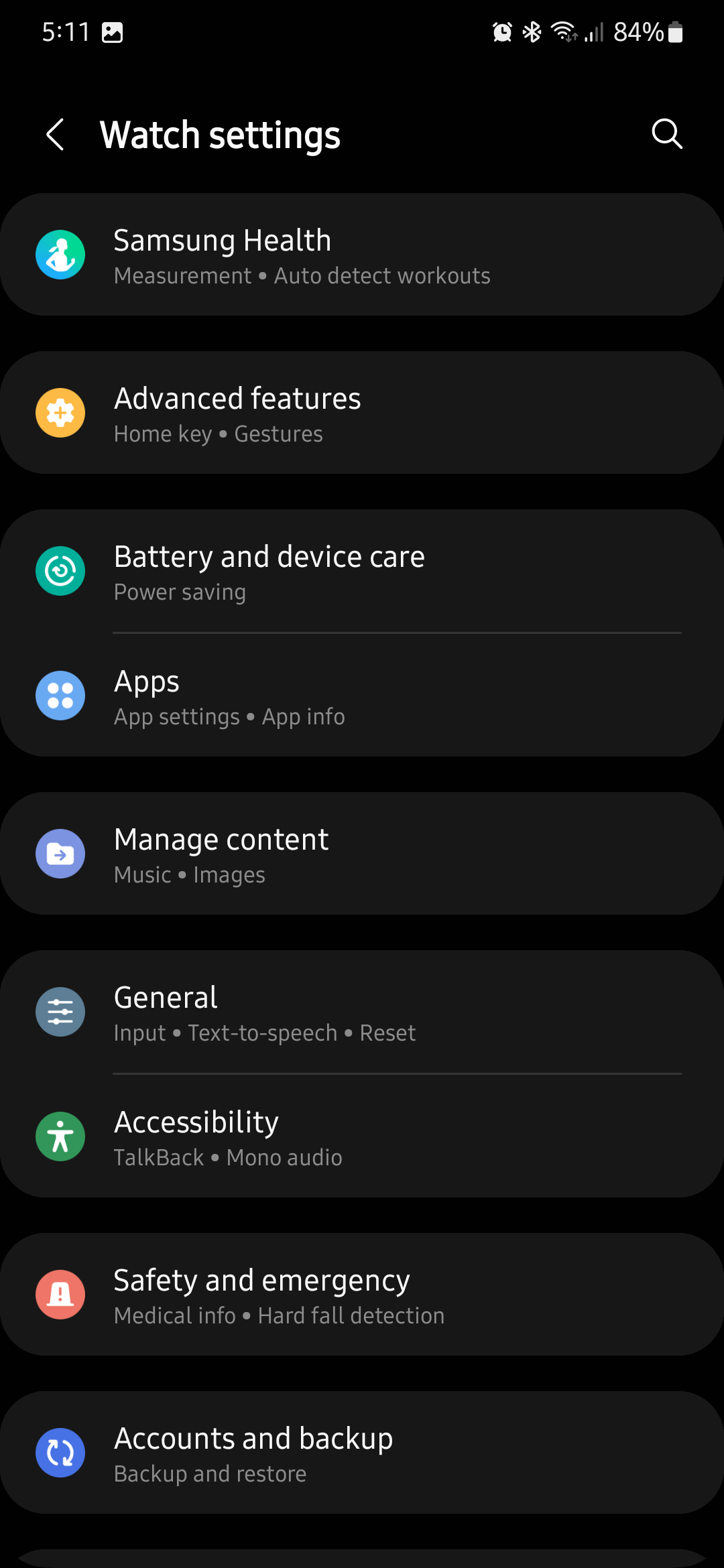This is a detailed screenshot of a smartphone's display set to dark mode. In the top left corner, the time is shown as 5:11, alongside the gallery icon. The top right corner features several status indicators, including the alarm clock icon, Bluetooth icon, Wi-Fi icon, network signal strength indicator, an 84% battery life indicator, and the battery icon itself.

Below these indicators, various sections related to device settings and configurations are visible. These sections include:

- **Watch Settings**
- **Samsung Health**, featuring options like Measurement, Auto Detects, and Workouts.
- **Advanced Features** such as Home Key Gestures.
- **Battery and Device Care**, with sub-options like Power Saving.
- Sections for **Apps**, including App Settings, App Info, and Management Content.
- **Music and Images** management.
- **General Input Text** for searching.
- Options related to **Reset** and **Accessibility**, featuring Talk Back and Mono Audio.
- **Safety and Emergency** settings, which cover Medical Info and Heart Fall Detection.
- **Accounts and Backup** features, including Backup and Restore.

Overall, this thorough description captures each detail visible in the screenshot and organizes the information in a structured manner.